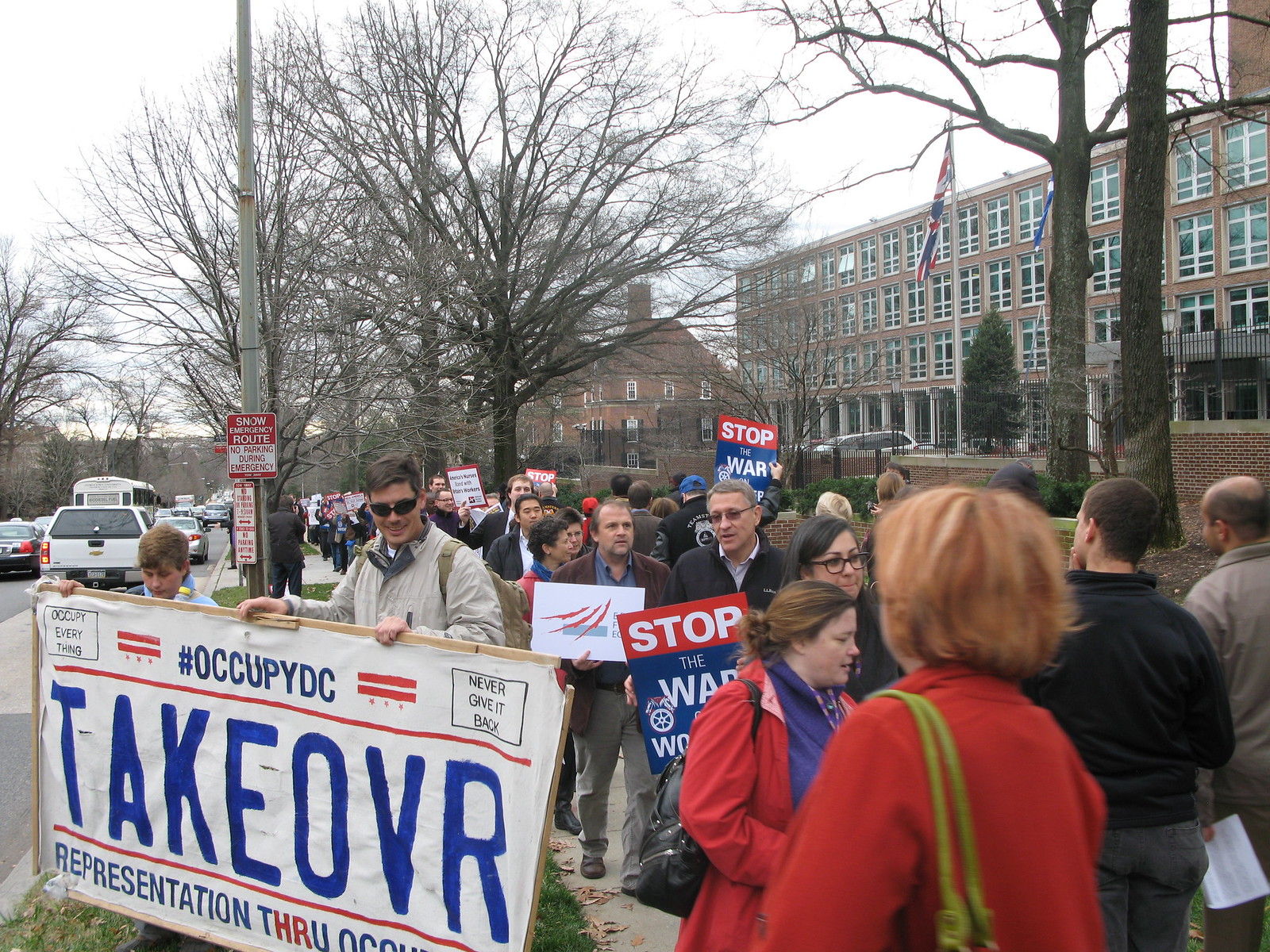The image depicts an overcast day with a white sky, where numerous people are gathered outside, participating in a protest. The bare trees, devoid of leaves, line the asphalt street to the left, which is bustling with moving vehicles and bordered by a grass strip. Prominent in the background are large brick buildings with numerous windows, and a government-like building with a flag. Various protestors, wearing light jackets, are crowded on the sidewalk, holding signs with messages such as "Stop the War" (displayed on a red and blue background) and "Occupy D.C. Takeover, Representation through ____," along with slogans like "Never Give It Back" and "Occupy Everything." Among the protestors, one person in a white jacket and dark glasses stands out, holding a sign resembling a license plate with blue text that reads "#OccupyDC Takeover." A woman with blonde hair, wearing a red jacket and a green-strapped shoulder bag, is noticeable at the bottom right. The scene also includes several poles with flags, an electrical or light pole, and people moving back and forth on the sidewalk, all contributing to the lively and dynamic atmosphere of the protest.